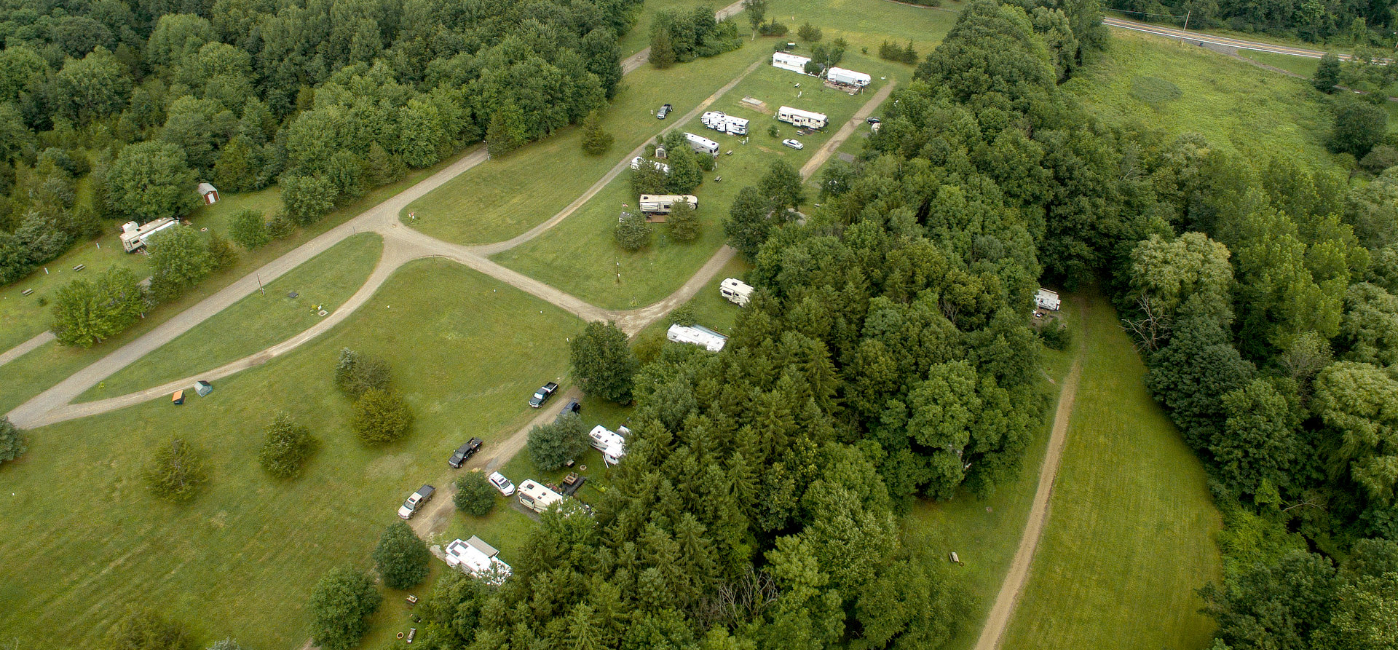The drone captures an aerial shot of a verdant field, intricately segmented by dense lines of trees and hedgerows forming various clearings. Winding through these sections are gravel and dirt driveways, some curving gracefully through the greenery. Central to the image is an RV camp, populated with numerous white RVs and accompanied by parked dark-colored cars. The layout features simple amenities such as campfire circles, indicating a casual, transient camping area rather than a permanent establishment with dedicated facilities. In the bottom right corner, a dirt road emerges from a clearing, leading to a solitary house. Another dirt road from a clearing off to the side extends into the photo, showcasing more RVs nestled among the trees. The entirety of the scene, bathed in mild light under a slightly overcast sky, suggests the photo was captured from approximately 200 feet above ground in the mid-afternoon. The rich greens of the trees contrast strikingly with the clear-cut grassy areas, creating a compelling, textured landscape.